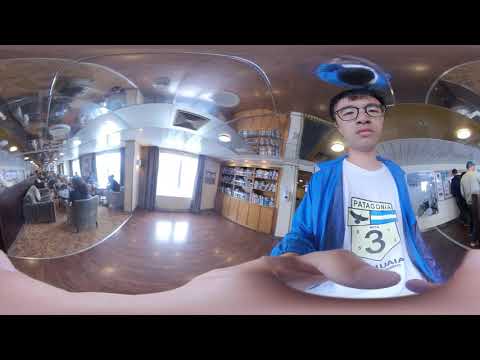A distorted panoramic image shows a man on the right side, appearing to take a selfie in what looks like a restaurant or airport lounge. The man, who appears to be Asian, has black hair and wears black-rimmed eyeglasses. He sports a serious, almost frowning expression, with his mouth shut. His outfit consists of a light blue, unbuttoned long-sleeved shirt draped over a white t-shirt with a yellow badge featuring the word "Patagonia," an image of a black eagle, and the number three.

Behind him, the floor is a smooth, shiny wood color, and there are sliding doors in the background with bright light shining through, creating reflections on the floor. The middle of the image features a wooden wall with shelves holding various items for sale. There's also an air vent visible on the ceiling, which is brown or copper-colored and somewhat reflective.

To the left, there is a seating area filled with patrons. The chairs are gray or green, and people are scattered among them, seated at tables. In the far-left background, another building section with brown carpeting is visible. On the far right, there is a convenience stand with a white wall and a line of people waiting to order.